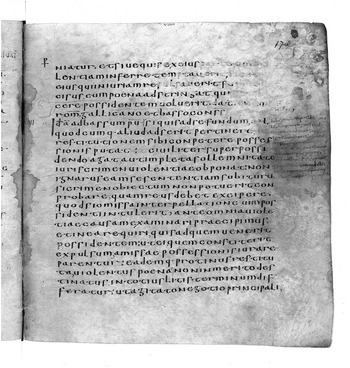This black-and-white photograph depicts a worn and ancient-looking page from a book. The left-hand page is partially cut off, with a visible fold line where the book has been opened repeatedly, accompanied by slight discoloration and staining. The right-hand side of the page is marred by circular water stains and dark spots, particularly near the upper corner. The page is covered in approximately 25 lines of text written in a romanized script that is unfamiliar and intricate, possibly penned with a quill. The text spans from the left to the right margins, which are about 3 inches from the edges of the page. The overall appearance of the page, enhanced by the monochrome shading, gives it a timeworn and weathered look suggestive of an ancient Latin manuscript.